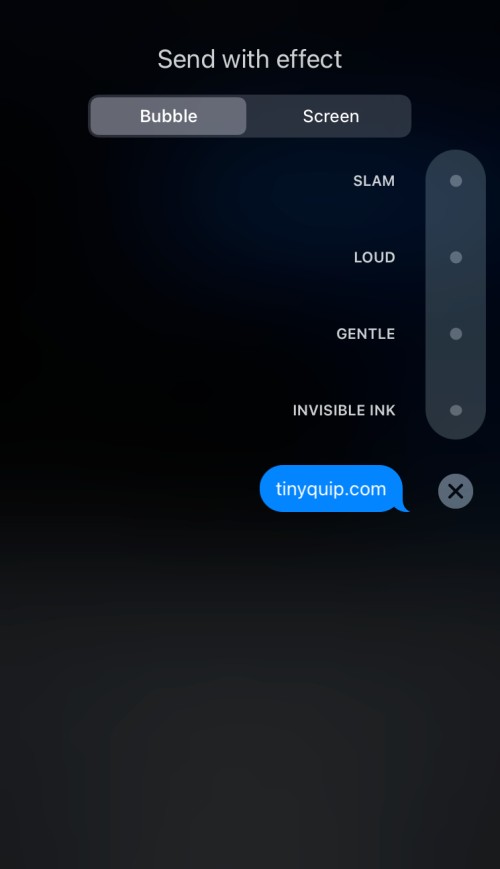This image is a vertically oriented screenshot from a cell phone, showcasing a particular setting within a messaging app. The primary color scheme is predominantly black, which slightly lightens towards the bottom, maintaining a dark theme overall. 

At the top of the screen, a grayish-white header reads "Send with effect." Directly beneath this header is a horizontal bar, divided into two sections: "Bubble" on the left, highlighted in a lighter gray, and "Screen" on the right, shown in a slightly dimmer white. The highlight around "Bubble" indicates that it is the currently selected option.

Below this bar, on the right side, a long, vertically aligned oval displays four selectable animation effects, each marked by a small dot. These options are listed as "Slam," "Loud," "Gentle," and "Invisible Ink."

Further down, a blue chat bubble containing the text "tinyquip.com" is accompanied by an 'X' icon, suggesting that this message is an example or template shown to illustrate how the selected text effect will appear in a conversation. 

The overall context of the screenshot indicates that the user is customizing the appearance and animation of their text messages within the app.